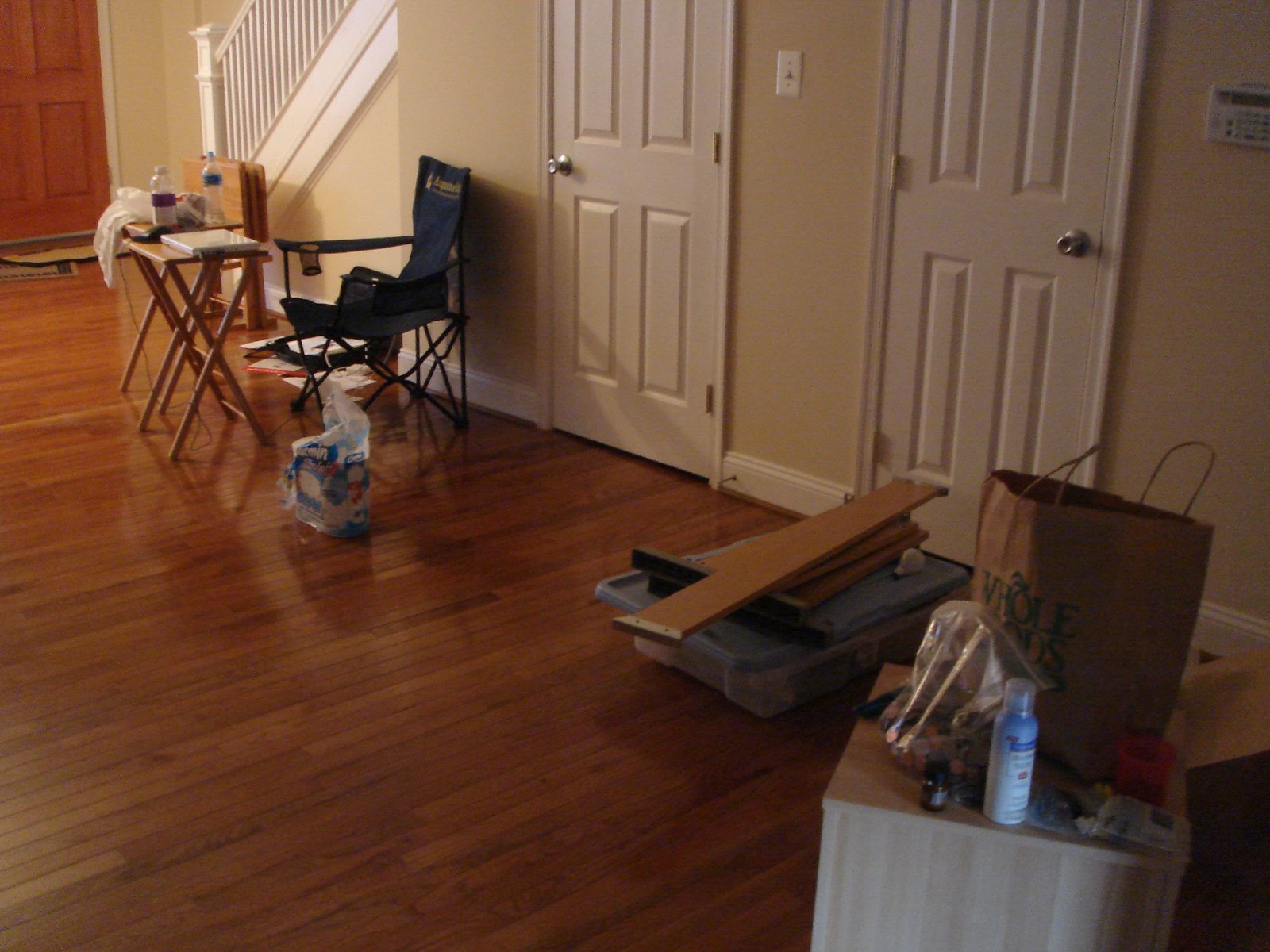The photograph appears to be taken in a cozy hallway of a home. In the upper left corner, a dark brown wooden door stands out against a yellowish wall. Adjacent to the door, a white wooden staircase ascends, drawing the eye upwards. The hallway's flooring is a rich dark brown wood, adding warmth to the space. 

Beneath the staircase, a neatly stacked set of three TV trays leans against the wall, with one tray open and holding a laptop computer and a plastic bottle. A black fold-up canvas camping chair is conveniently positioned nearby, suggesting a casual, makeshift workspace. 

Next to the chair, a plastic bag rests on the floor, possibly containing a bottle of water. The yellowish wall behind the chair hosts two white doors with round silver handles, and between them, a single white light switch is mounted.

In the bottom right-hand corner, a small square wooden table holds a paper sack and a blue bottle of sunscreen, adding a touch of everyday life to the scene. The overall composition is a detailed snapshot of a functional and lived-in space.